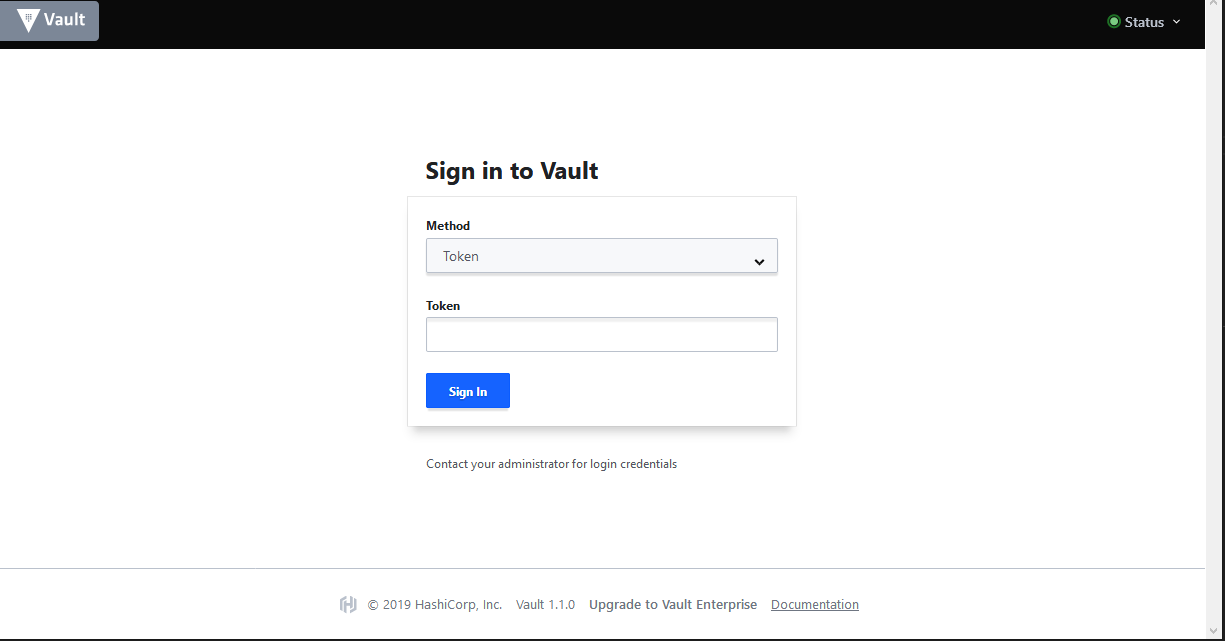This is a detailed caption describing a screenshot of a webpage:

The screenshot displays a webpage with the title "Vaults" located in the upper left-hand corner. Adjacent to the title is a home icon, which is depicted in a medium gray color. Next to the icon, there is a white equilateral triangle pointing downward, and the text "Vault" with a capital "V" is displayed beside it. This entire section is situated within a black bar that spans the top of the screen.

In the upper right-hand corner of this black bar, a green circle is featured, with the word "Status" beside it and a downward-pointing chevron. 

The majority of the webpage below this banner is predominantly white and largely empty. However, a sign-in box is prominently centered on the page. The box is titled "Sign in to Vaults," with "Vaults" in bold text. Below this title, users are instructed to select their sign-in method and provide their token. The sign-in box contains input fields for these details and a blue button for submission. An advisory note below the button reads, "Contact your administrator for login credentials."

At the bottom of the webpage, a footer spans the width of the screen. This footer contains the text: "2019 HashCorp Inc., Vault 1.1.0. Upgrade to Vault Enterprise," along with a link labeled "documentation." All text within the footer is rendered in the same medium gray color as the home icon.